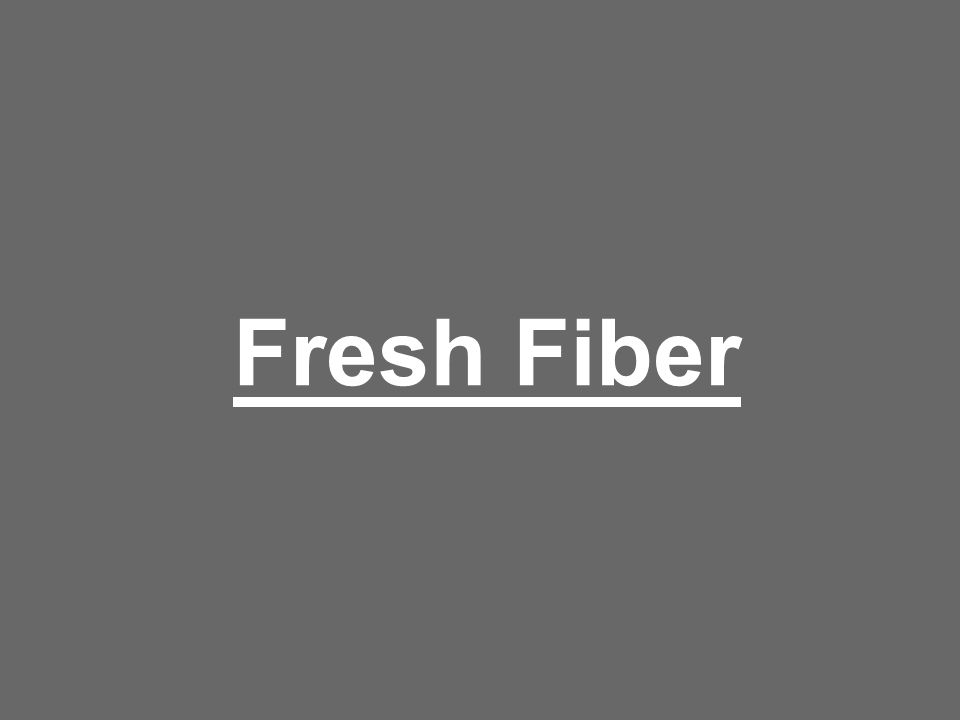The poster features a horizontally rectangular shape with a dark gray background, which is smooth and solid in color. Positioned in the direct center of this poster are the words "FRESH FIBER" in large, bold white letters, written in a Sans Serif font. Both 'F's are capitalized, and there is slight spacing between each letter. Directly underneath the text is a thin, horizontal white line that perfectly aligns with the length of the two words, acting as an underline. The poster is simple and devoid of any additional images, text, shadows, or effects, giving it a minimalist and clean look.